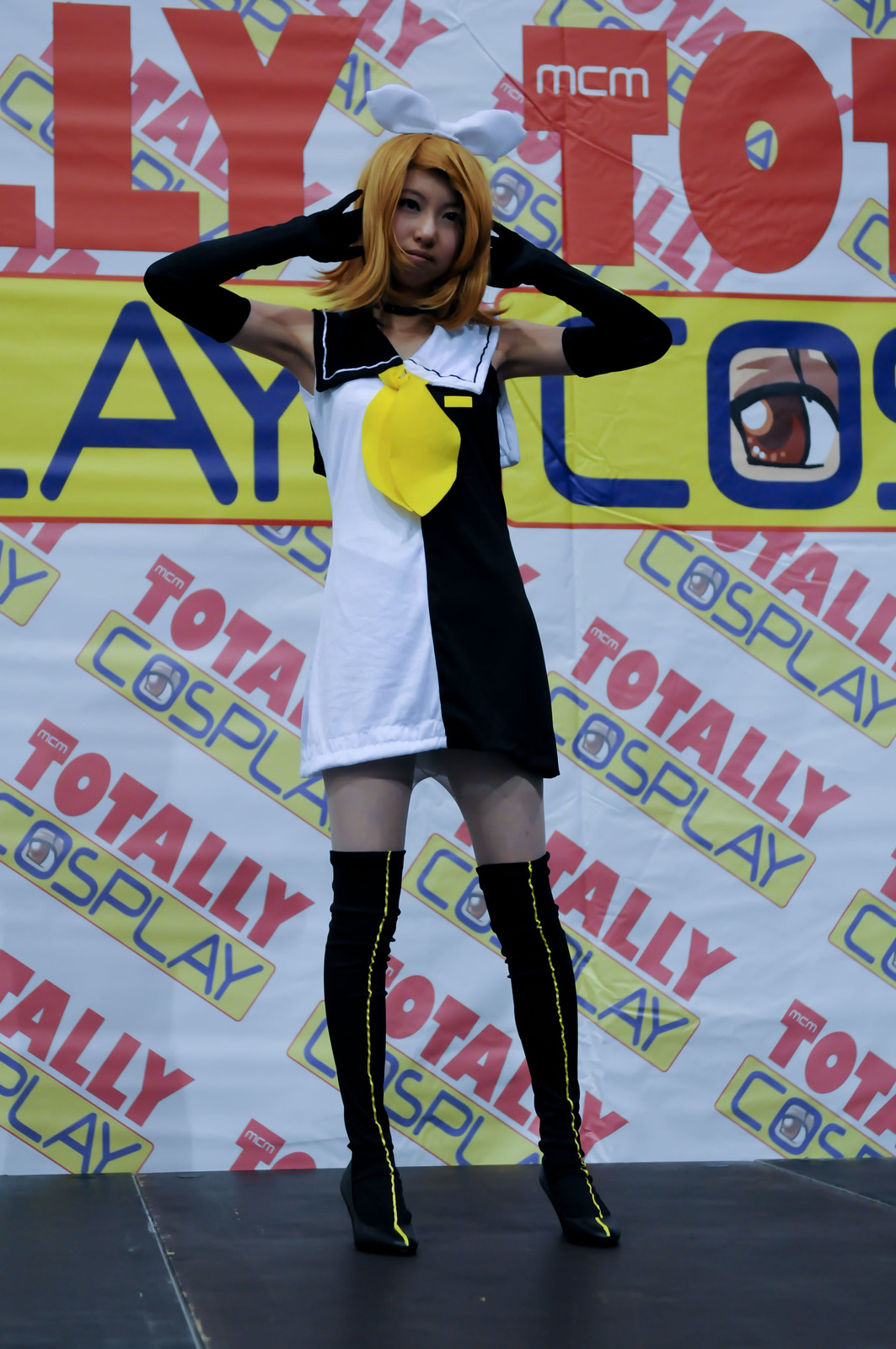In the photograph, there is a young, very thin Asian woman standing confidently as she showcases her cosplay outfit in front of a large "Totally Cosplay" banner. She is dressed in a striking black and white sleeveless dress that transitions at the center, with black on the right side and white on the left. The dress, adorned with a large yellow tie-like ribbon and a matching yellow name tag on her left chest, compliments her elaborate attire. She wears thigh-high black boots with thin yellow stripes running vertically down the front and long black gloves that extend past her elbows. Her hair, a vibrant blend of orange and reddish hues, cascades down to her shoulders. The banner behind her features diagonal text with "Totally" in red and "Cosplay" in blue within a yellow rectangular bar, emphasizing the cosplay event she is participating in. Her pose, with arms bent and hands behind her head, adds to the dynamic and energetic feel of the image.